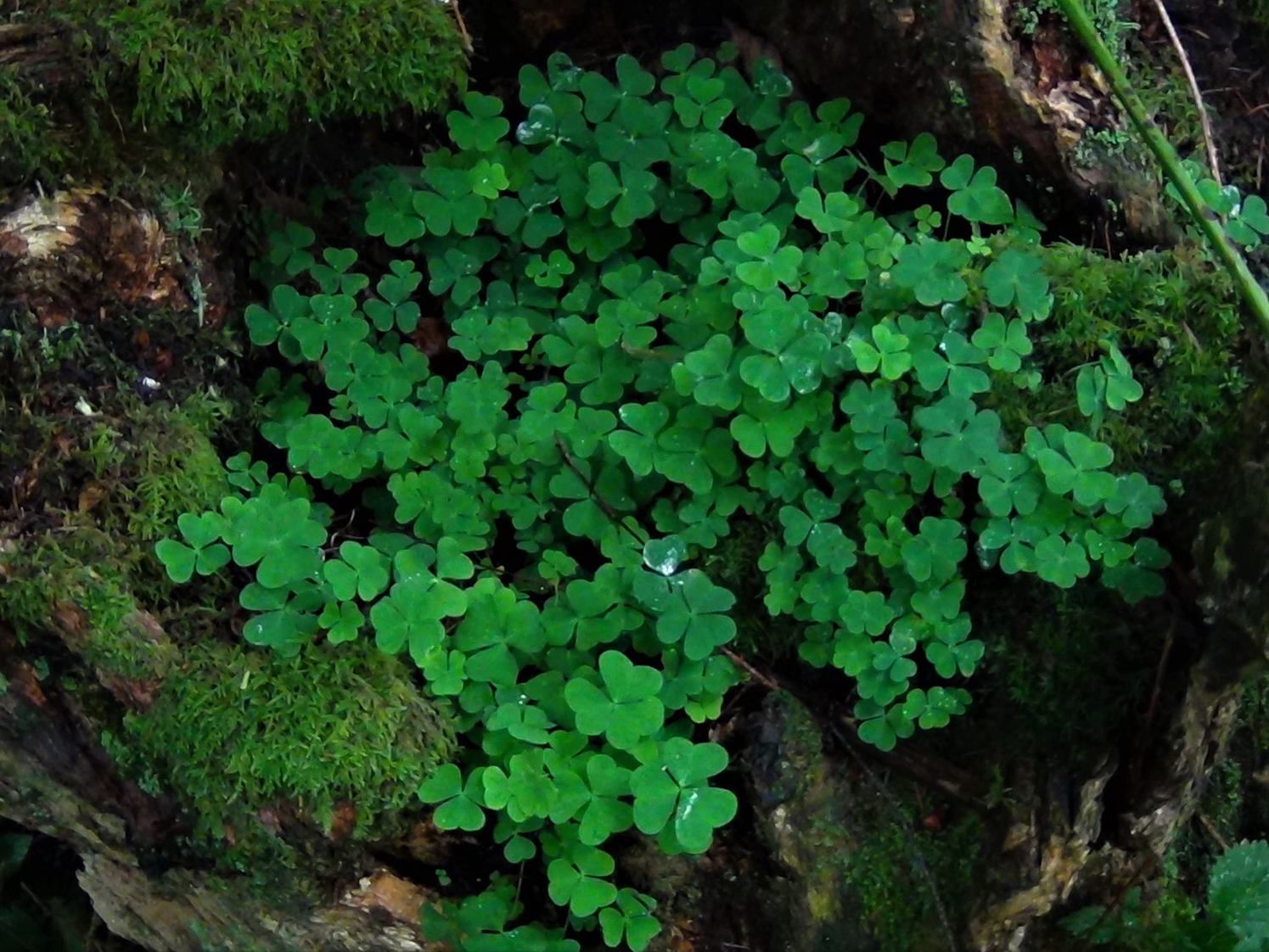The image captures a vibrant cluster of bright green clovers, predominantly three-leaved, growing out of a depression in a tree trunk. This natural setting features moss with hues of green and brown, visible in the lower left and upper left corners of the frame. The background is complemented by a tree branch in the upper right corner, showcasing a notable cavity or hole. The tree's texture and the shiny appearance of the clovers, potentially due to recent rain, add to the rich, detailed ambiance of the photograph.